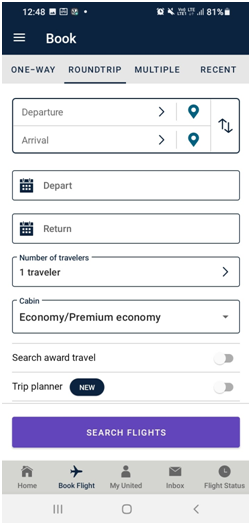The image showcases a mobile phone screen displaying a flight booking page. At the top of the screen, the title "Book" is prominently featured, with the "Round Trip" option underlined in the trip selection section below, where choices for "One Way," "Round Trip," "Multiple," and "Recent" trips are available. The departure and arrival fields, equipped with dropdown menus and location pins, are ready for user input. Below these fields, two rectangular buttons labeled "Depart" and "Return" are visible, each accompanied by a calendar icon on the left side.

Scrolling further down, the screen indicates the "Number of Travelers," which has been set to one traveler. The cabin class is specified as "Economy/Premium Economy." Following this, the screen shows options for "Search Award Travel" and "Trip Planner," each marked with a "New" tag. However, both features are toggled off, as indicated by the sliders at the end of their respective rows.

At the bottom of the booking form, a prominent purplish-blue button labeled "Search Flights" invites users to initiate their search. The very bottom of the screen features navigation icons for "Home," "Book Flights," "My United," "Inbox," and "Flight Status."